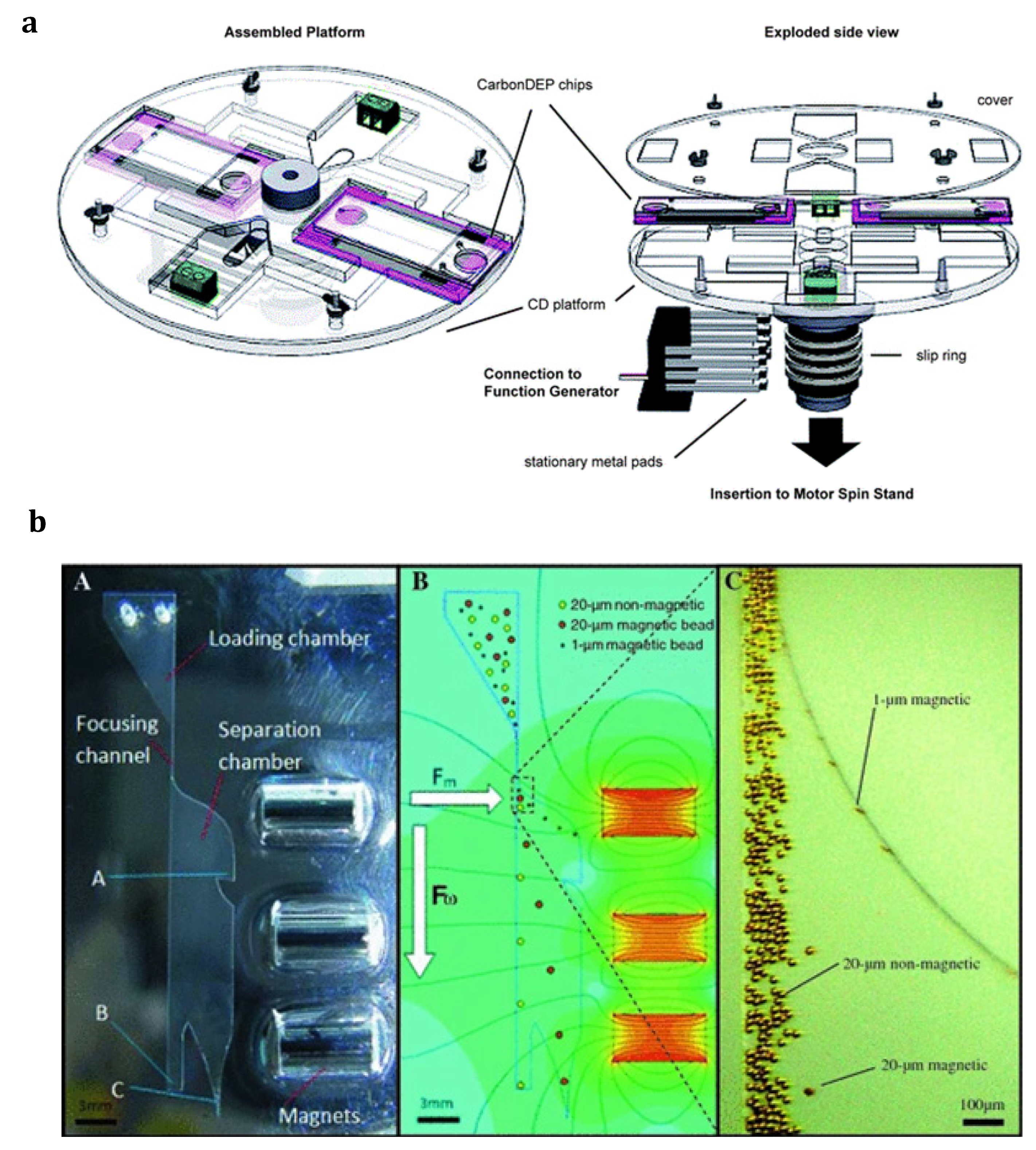The image presents a detailed engineering schematic showcasing a complex piece of technology. In the top left corner, a labeled circle reads "assembled platform," accompanied by labels such as "carbon DEP chips," "exploded side view," "cover," "CD platform," "connection to function generator," "stationary metal pads," "insertion to motor spin stand," and "slip rank." Adjacent to this, two circles—one of which is blown out—depict some kind of spinning mechanism or assembly. Below, the diagram illustrates three separate images: the first is predominantly blue, outlining a "focusing channel," "loading chamber," "separation chamber," and "magnets"; the adjacent image is green with orange rectangles and indicates "20 UM non-magnetic"; while another green-toned image displays yellowish-green balls. This meticulous chart blends detailed textual labels, intricate schematics, and what seem to be microscopic images, providing a comprehensive look into the internal components and operation of this sophisticated device.